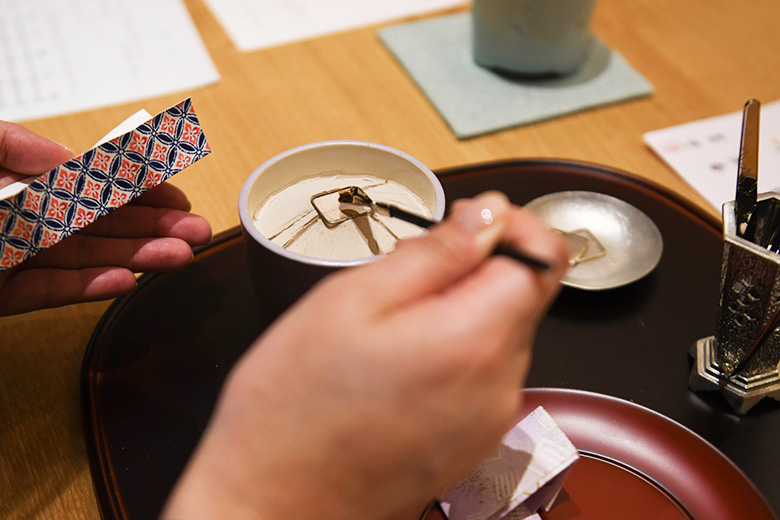The image captures a detailed scene of someone engaged in a Japanese incense ceremony. The focal point is a pair of hands, gently manipulating the tools of the craft. In the left corner, the left hand delicately holds a piece of intricately designed red, white, and black paper, with circular patterns meshed together. The right hand clutches a long black-necked tool with a silver base, dipping it into a small bowl on the table. Adjacent to this bowl, another small bowl sits to the right, and a red plate is situated in the lower right corner. The table is adorned with additional items including post-it notes and what appears to be a coaster with a glass. The wood-grain table and the arrangement of various colored objects—blue, red, silver, gold, light green, black, peach, and light brown—create a rich, textured background. The setting is intimate, displaying the meticulous nature of the incense preparation, with shallow dishes and tools arranged carefully, emphasizing the ceremonial aspect of the experience.